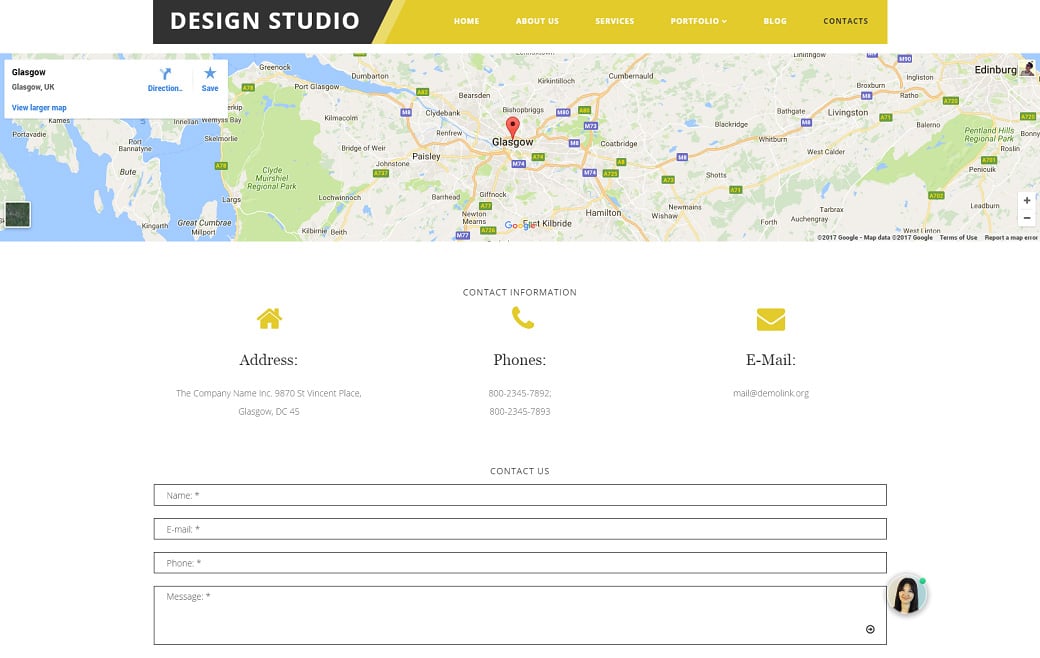This image is a horizontal screenshot of a webpage from a design studio. The top banner of the webpage is black with white text reading "Design Studio," and has a yellow section on the right listing navigation links: Home, About Us, Services, Portfolio, Blog, and Contacts. The banner does not extend fully to the edges of the screenshot, leaving white spaces on both sides.

Below the banner is a wide horizontal strip featuring a map of Scotland. A location icon highlights the city of Glasgow, while the city of Edinburgh, labeled at the top-right corner, has a small profile picture adjacent to its label. The map details various routes, areas, natural features, and bodies of water. A white pop-up box at the top left of the map provides options to save the map, view a larger version, and select map directions.

Beneath the map, a large white section displays icons and details for contact information. The address is listed alongside two phone numbers and an email address. Following this section is a "Contact Us" form, which includes fields for the user's name, email, phone number, and message. To the right of the form's text boxes, a small profile picture of a woman features a green dot to the right of her head, indicating online availability or presence.